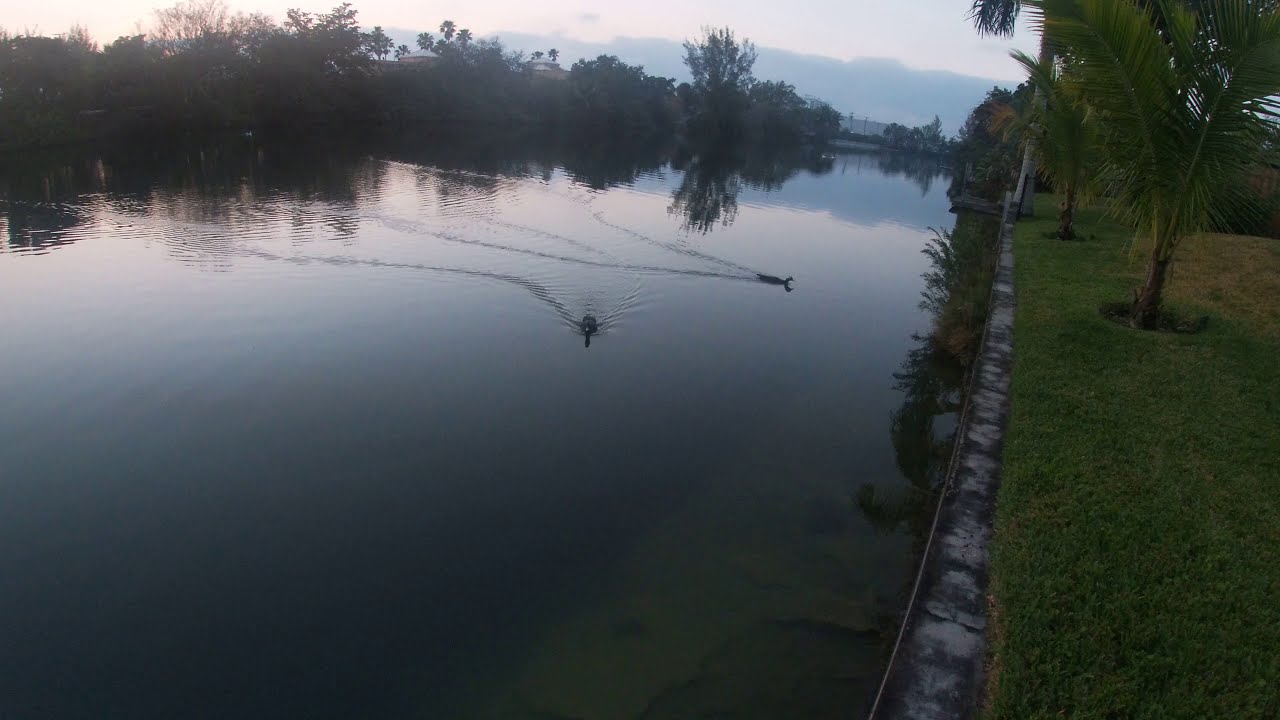In this serene image, a body of water, likely a man-made pond or canal, is bordered by a cement or brick wall on the right, separating it from a stretch of land. The waterway showcases two ducks swimming gracefully, their paths traced by faint ripples left behind them. The landscape on the right side features patches of green grass interspersed with areas of drought, and young palm trees, approximately ten years old, sprouting from the ground. Behind the ducks, in the distance, trees and shrubs poke out from the banks of the water, adding to the natural ambiance. The scene is set against a backdrop of hills and a dusky sky, which casts a subtle gray hue over the tranquil panorama.